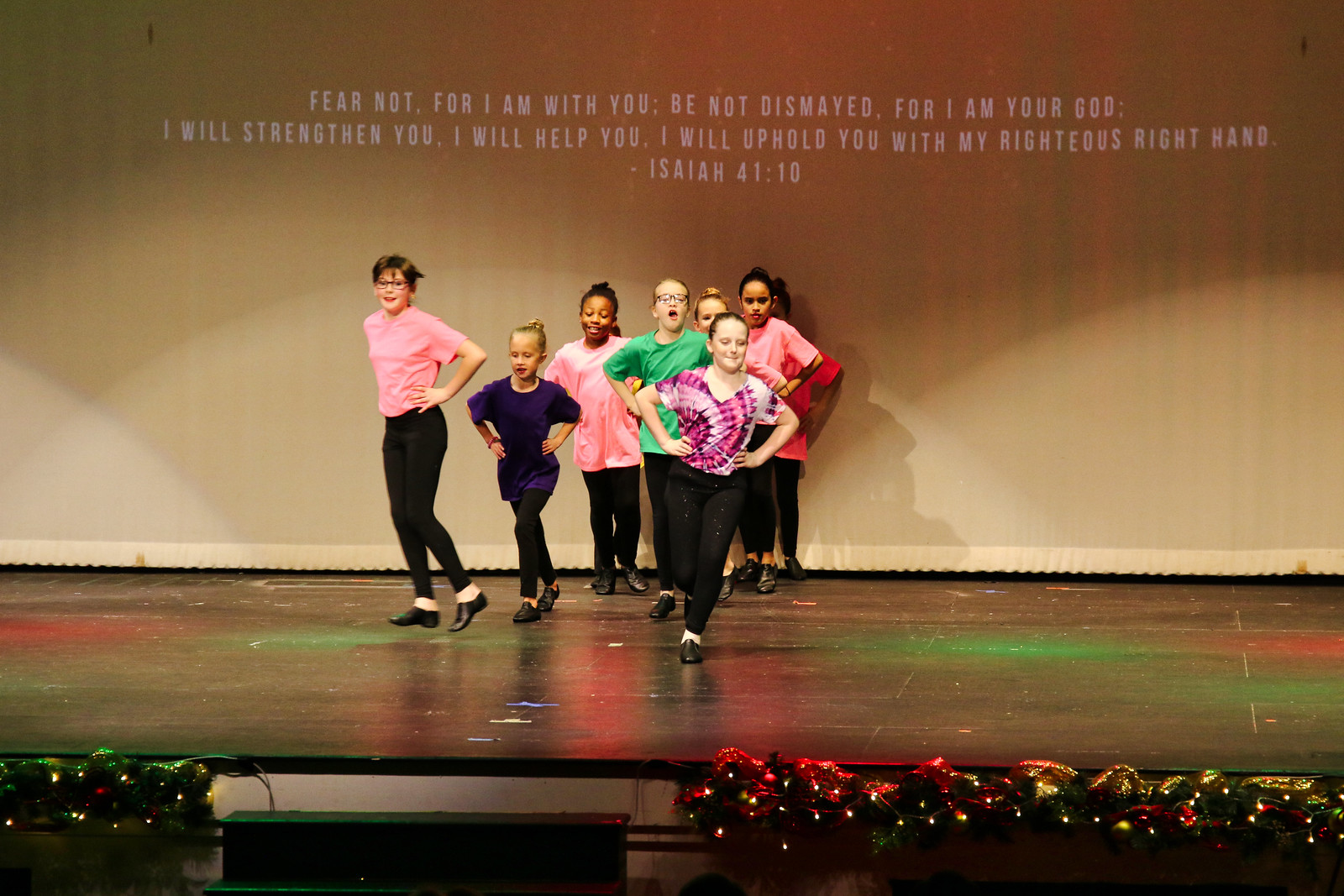This detailed photograph captures a lively scene of young girls performing on a stage, framed in a horizontal, landscape view. The girls, who appear to be between 5 and 11 years old, are dressed in bright, colorful attire, each wearing short-sleeved shirts in an array of hues such as pink, red, green, navy, and even a maroon tie-dye design. Complementing their vibrant tops, they sport black pants and tap shoes, ready for a dance performance on the wooden floor beneath them.

The setting is festive and vivid, with red and green stage lights illuminating the scene. Christmas lights adorn the front edge of the stage, adding to the cheerful ambiance. Behind the girls, a tan or white curtain backdrop gracefully hangs, serving as the perfect canvas for an inspiring quote that is prominently displayed above them. The text reads: "Fear not, for I am with you; be not dismayed, for I am your God. I will strengthen you, I will help you, I will uphold you with my righteous right hand. Isaiah 41:10."

Centered and clearly visible in the photograph, the quote complements the vibrant and joyful energy of the girls' performance, creating a heartwarming and dynamic snapshot.